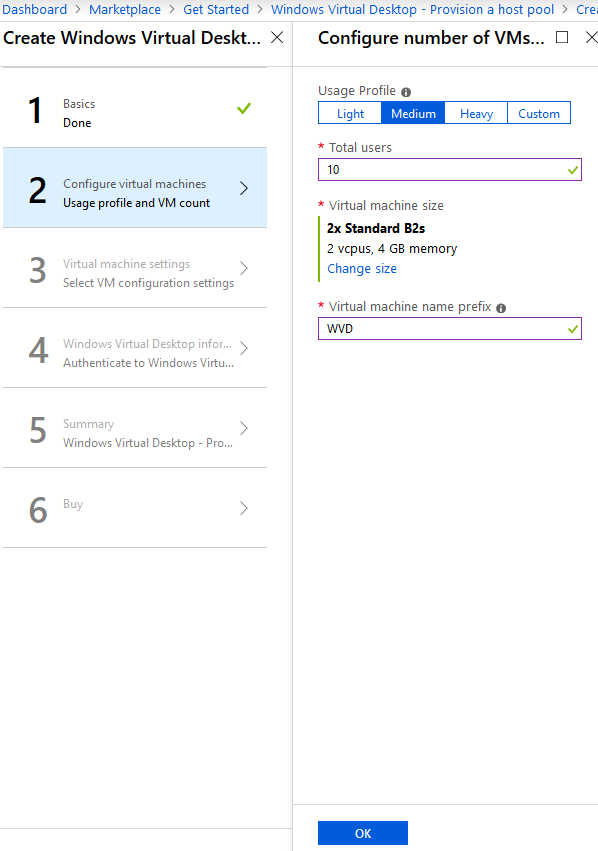This image displays a screenshot of a configuration interface for setting up a Windows Virtual Desktop via a web dashboard. At the top of the interface, the title bar reads "Dashboard Marketplace Get Started Windows Virtual Desktop - Provision a Host Pool." Below this, a multi-step configuration process is visible.

Step 1, labeled "Basics," has been completed, and the image highlights Step 2, which is "Configure Virtual Machine." This step includes settings for "Usage Profile" and "VM Count." On the right side of the interface, a menu allows users to specify the number of virtual machines (VMs) needed. Within this menu, the "Usage Profile" dropdown offers options such as "Light," "Medium," "Heavy," and "Custom." Below this, the current configuration is set to a total of 10 VMs.

In the "Virtual Machine Size" section, "2x Standard B52s" is selected, featuring specifications of "2 vCPUs" and "4 GB memory." A clickable "Change Size" option suggests the ability to select different VM configurations.

Further down, the "Virtual Machine Name Prefix" field is populated with "WVD," likely abbreviating "Windows Virtual Desktop."

The subsequent steps in the configuration process are briefly visible, including:

- Step 3: "Virtual Machine Settings"
- Step 4: "Windows Virtual Desktop Information"
- Step 5: "Summary"
- Step 6: "Buy"

This screenshot appears to guide users through the process of customizing and potentially purchasing a Windows Virtual Desktop setup.